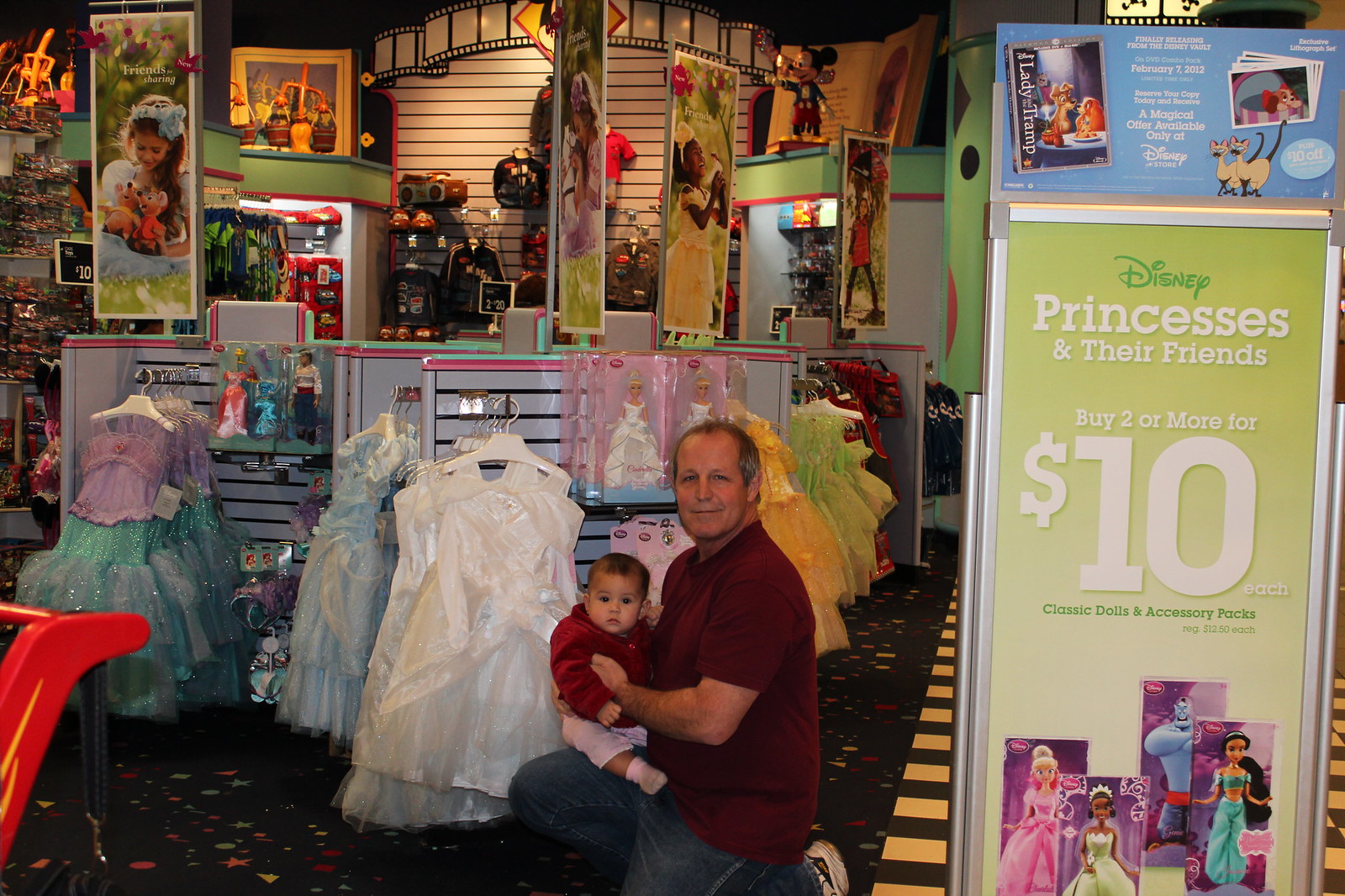In the vibrant Disney store, a joyful older man, likely in his fifties or sixties, kneels with a baby, who appears to be about one or two years old, on his knee. Both are facing the camera with the man smiling widely while the baby gazes curiously at the lens. The man, dressed in a red shirt, blue jeans, and white shoes, holds the baby in a red jacket, pink pants, and matching pink shoes.

The store around them is a whimsical wonderland of Disney magic. Behind them, an array of colorful Disney princess dresses, including those of Cinderella, Ariel, Snow White, and Jasmine, fills the space. The background reveals shelves and racks lined with dolls, toys, and various themed merchandise, all meticulously arranged.

A prominent banner advertises a special deal: "Disney princess and their friends. Buy two or more for $10 classic doll accessory packs." This signage is part of a lively shopping environment, which features vibrant carpeting designed to look like colorful confetti, and decorative elements that nod to Disney’s cinematic history, such as Mickey Mouse and the Mops from Fantasia, as well as backlit marquee lighting styled to resemble a movie film reel.

In the foreground, the detailed display and signage ensure that every aspect of the store exudes a festive and animated atmosphere, perfect for creating cherished memories.